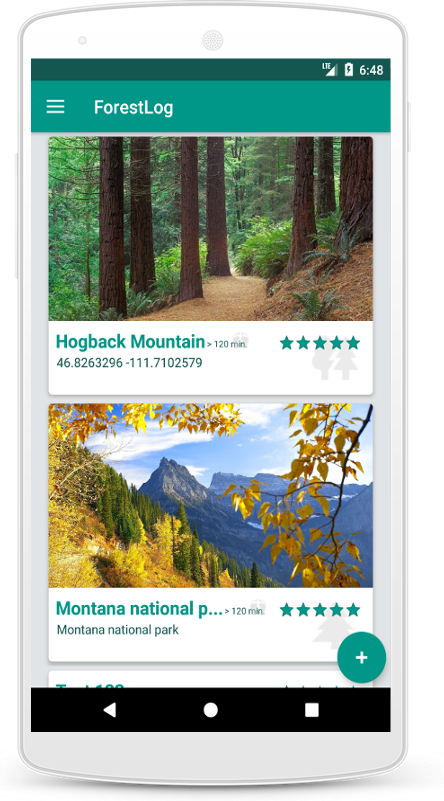This vertical rectangular image depicts a cell phone with a white top and bottom edge, as well as a white border encircling the device. At the top of the screen is a thin horizontal area colored hunter green, which prominently displays the time "6:48" in white font on the upper right corner next to an almost full battery icon. Below this section, there's a brighter green horizontal strip where the phrase "ForestLog" is written in white font, with capitalized "F" and "L". Beneath that, the main content begins with an image of various tree trunks without leaves, suggesting a path in a forest with additional trees visible in the background and a dirt path winding through the scene. 

Immediately below the image, in a white section, "Hogback Mountain" is emblazoned in bright green font, accompanied by a set of five green star icons indicating a rating. Further down, another image showcases a picturesque view of mountains under a blue sky dotted with white clouds. In the foreground, green trees are visible, with yellow leaves hanging from branches on the right and left sides. Under this image, the text "Montana National" is displayed in green font, followed by capital letter "P" and five green stars, with "Montana National Park" written underneath. This detailed layout suggests a digital interface related to a nature or travel application highlighting picturesque locations and their ratings.